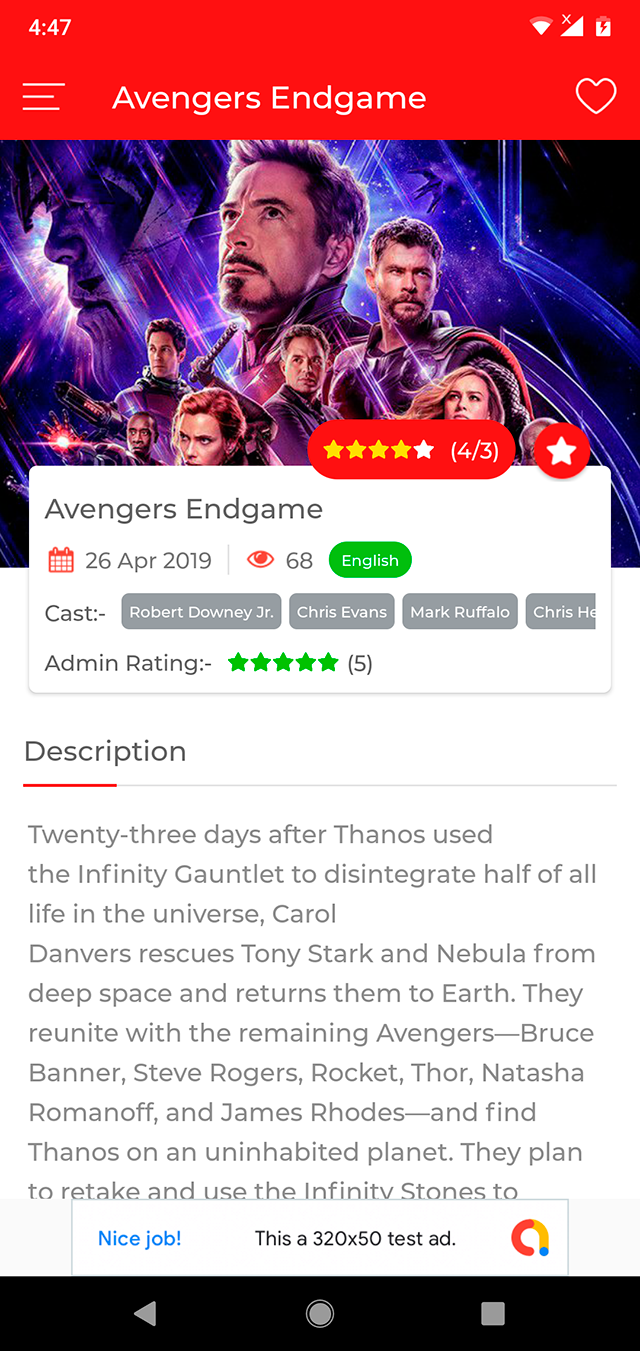Screenshot from *Avengers: Endgame*: The image features Robert Downey Jr., portraying Tony Stark, with his signature brown hair, brown eyes, mustache, and goatee. He appears to be around 45 years old. Standing next to him is another male character, with several more recognizable actors and actresses in the background, embodying some of Marvel's most iconic heroes. The text on the screen narrates a pivotal moment, 23 days post-Thanos's catastrophic use of the Infinity Gauntlet to wipe out half of all life in the universe. It details how Carol Danvers, also known as Captain Marvel, rescues Tony Stark and Nebula from the depths of space and returns them to Earth. Upon their return, they reunite with the remaining Avengers: Bruce Banner (Hulk), Steve Rogers (Captain America), Rocket, Thor, Natasha Romanoff (Black Widow), and James Rhodes (War Machine). Together, they locate Thanos on an isolated planet, strategizing to reclaim and utilize the Infinity Stones. Additionally, a small pop-up ad at the bottom of the screen reads, "Nice Job. This is a 320x50 test ad."